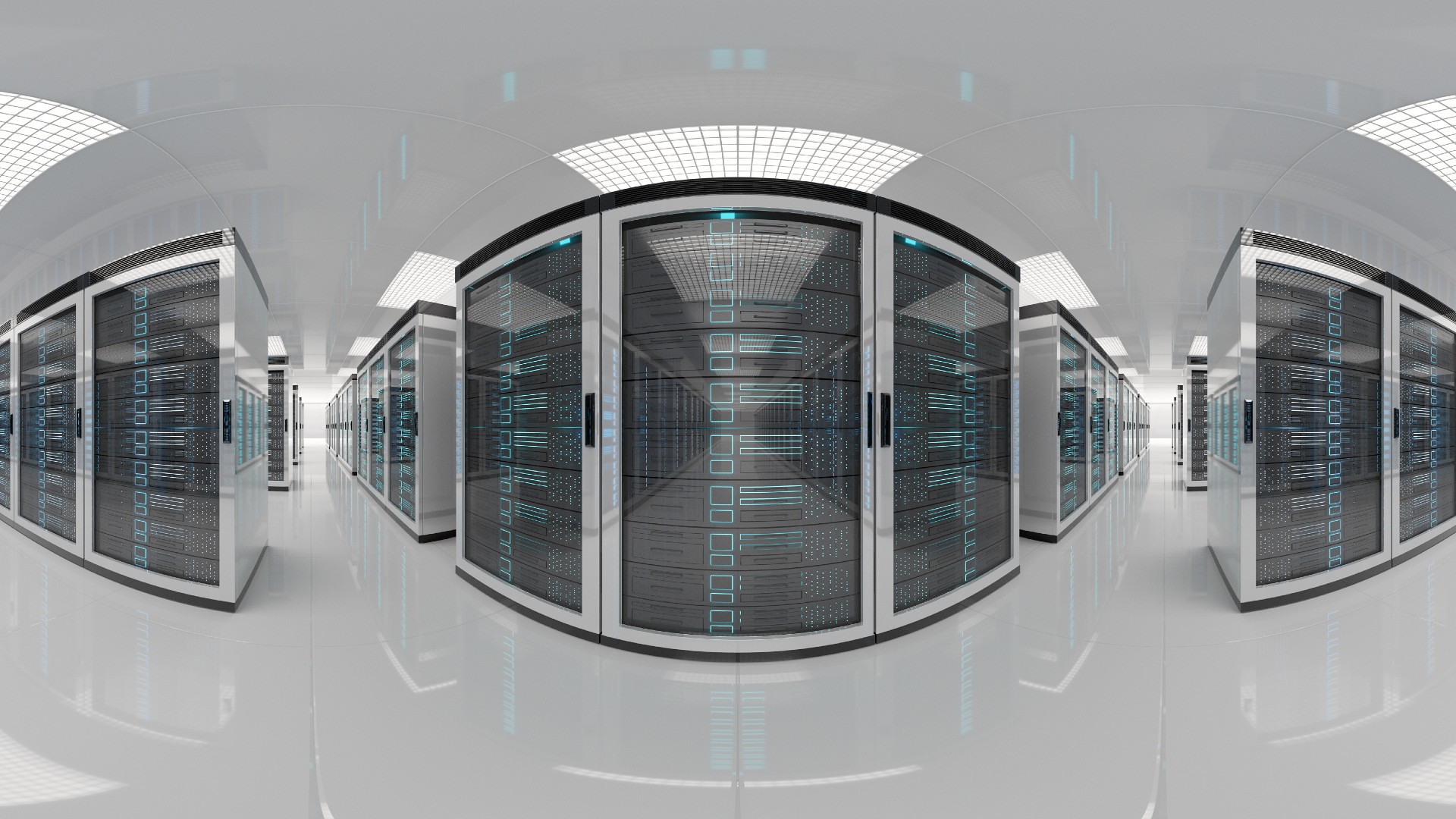The image depicts a sleek, ultra-modern indoor space, possibly a computer-generated rendering of a large database room. The room has a soft gray background and features glossy, reflective gray floors that exude a pristine shine. The ceiling is adorned with an array of white grid-marked lights, contributing to the room's bright, clean atmosphere. 

Dominating the room are substantial black structures, including several large cabinets with multiple stacked hard drives, illuminated by blue lights. These cabinets line the central area and are flanked by similar units on both sides, creating rows and aisles that extend deep into the background, facilitating easy navigation. The overall ambiance suggests an echoic, immaculate environment.